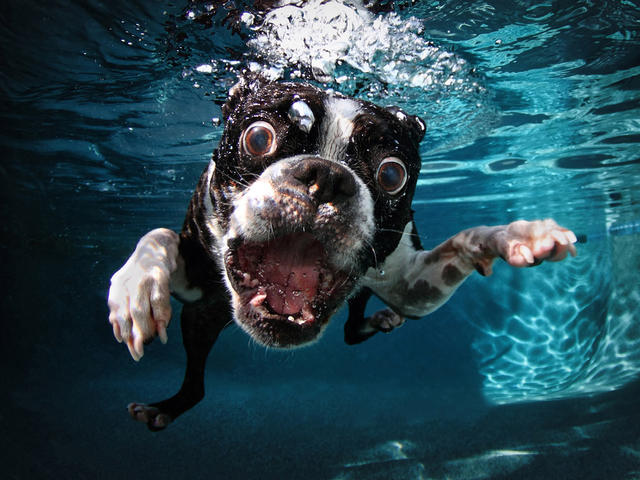A high-quality, comical image features a Boston Terrier underwater, freshly submerged after an enthusiastic dive. The dog, with striking black and white fur, exhibits an expressive, terrified face, staring straight into the camera. Its mouth is agape, showcasing its teeth, while its large, brown eyes are wide open, the whites clearly visible against the dark pupils. Residing in what seems to be a backyard swimming pool with dark blue walls and shimmering reflections, the water glitters in various shades of blue. Small bubbles trail from the dog's nose, alongside larger bubbles above its head, indicating its recent plunge. The terrier's paws, prominently featuring white and grey spotting, thrust forward in a swimming motion, with the black legs visible against the aqua-tinted, crystal-clear water. The scene captures a blend of the dog's panic and excitement, framed by a vivid underwater environment.